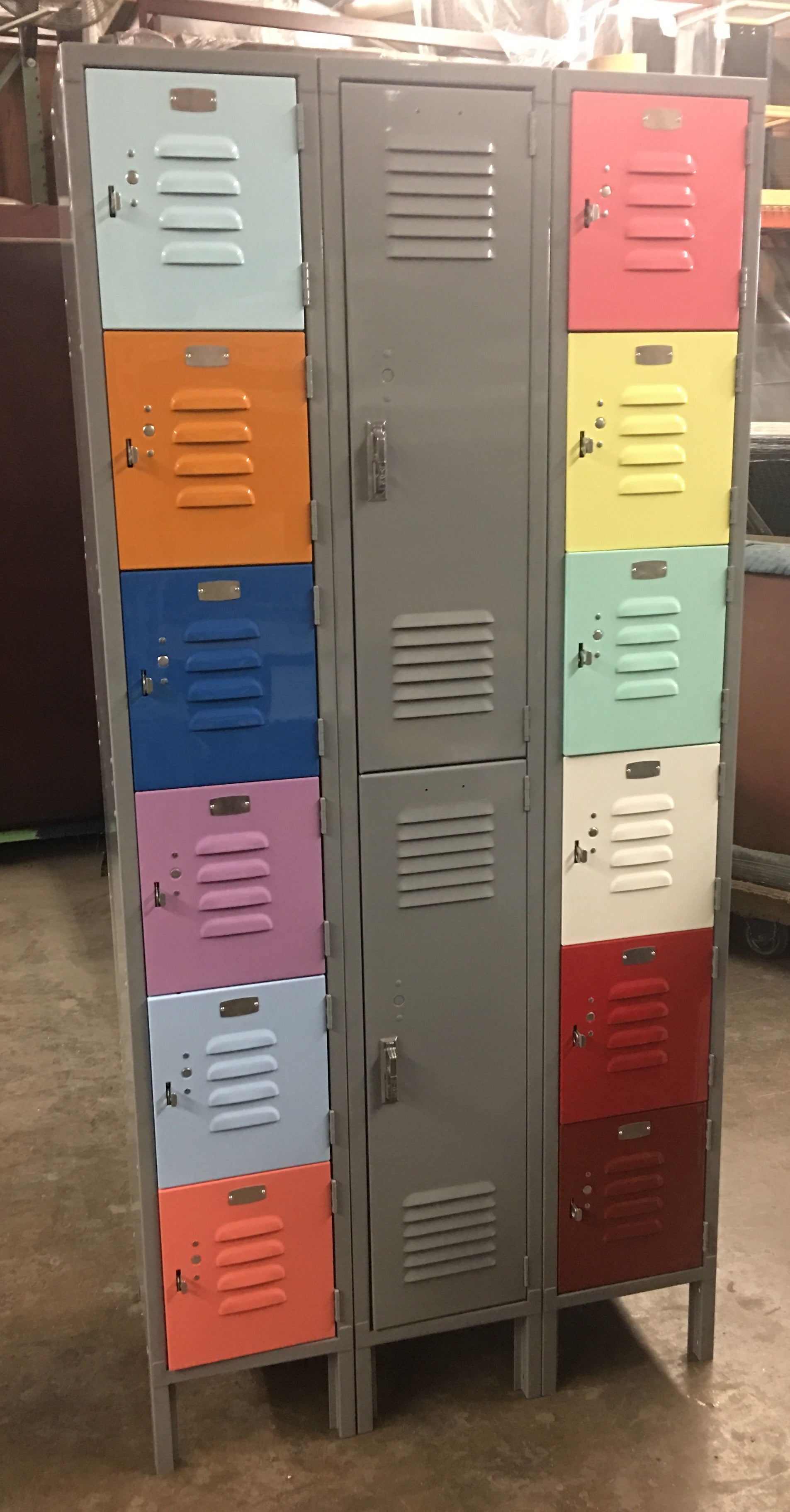In this image, there is a series of connected lockers arranged in two horizontal rows of three, making a total of six lockers. Each locker has a distinct color and pattern. 

Starting from the bottom left, the first locker features a salmon-pink-orange color, followed by a light blue locker in the middle, and a light purple locker on the right. In the top row, the first locker is dark blue, the middle locker is orange, and the right locker is light blue.

On the bottom-right section, the first locker is dark red-brown. Above this locker is one with a red square design, followed by another locker with a white square design. The top right locker consists of patterns in light blue, light yellow, and pink.

The flooring around the lockers is gray, and the background wall on the left side of the image is dark brown. Part of the ceiling is also visible in the picture, adding to the overall context of the space.